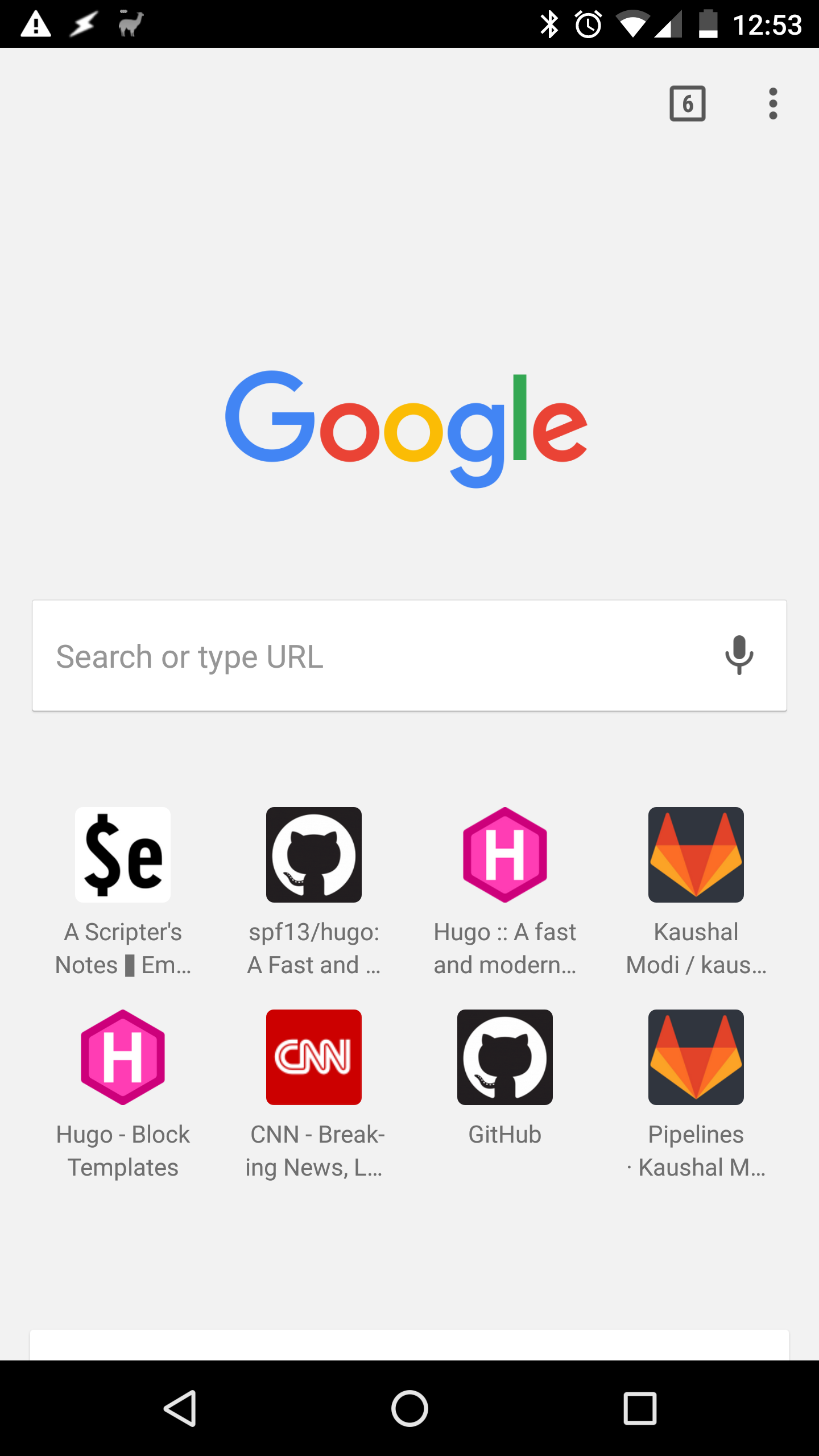This image features a smartphone screen set against a gray background. The phone screen itself displays the following elements in detail:

- At the top of the screen is the phone's UI with various status icons. These include:
  - A warning icon
  - A thunderbolt icon
  - A llama icon
  - The Bluetooth icon
  - An alarm clock icon
  - The WiFi strength icon
  - A battery icon indicating a low charge
  - The time, displayed as 12:53

- Below the status bar, the browser interface is visible. Starting from the top right corner, there's a small number "6" next to three vertical dots (likely a menu button).

- Below these icons is the Google search bar, prompting "search or type URL" with a microphone icon positioned to its right.

- Under the search bar, there are several website thumbnails and icons arranged in a grid. Each has a brief description:
  - An icon noted as "scriptor's note"
  - A website titled "SE" with the background showing "SPF 13 / Hugo" and a cat silhouette icon
  - Another Hugo-related site titled "Hugo, a fast and modern," featuring a purple "H" hexagon icon
  - "Kaushal Modi" presented with a pixelated, Art Deco-style fox head
  - "Hugo block templates" again with the same purple "H" hexagon icon from before
  - The CNN website with its recognizable red CNN logo
  - GitHub displayed with the silhouetted cat icon
  - "Pipelines" accompanied by the fox-like icon previously seen with Kaushal Modi

- At the bottom of the screen, you can see the standard Android navigation buttons:
  - The back button (triangle)
  - The home button (circle)
  - The recent apps button (square)

The composition of the screen is clear and detailed, highlighting both the common functional icons and the specific accessible websites.